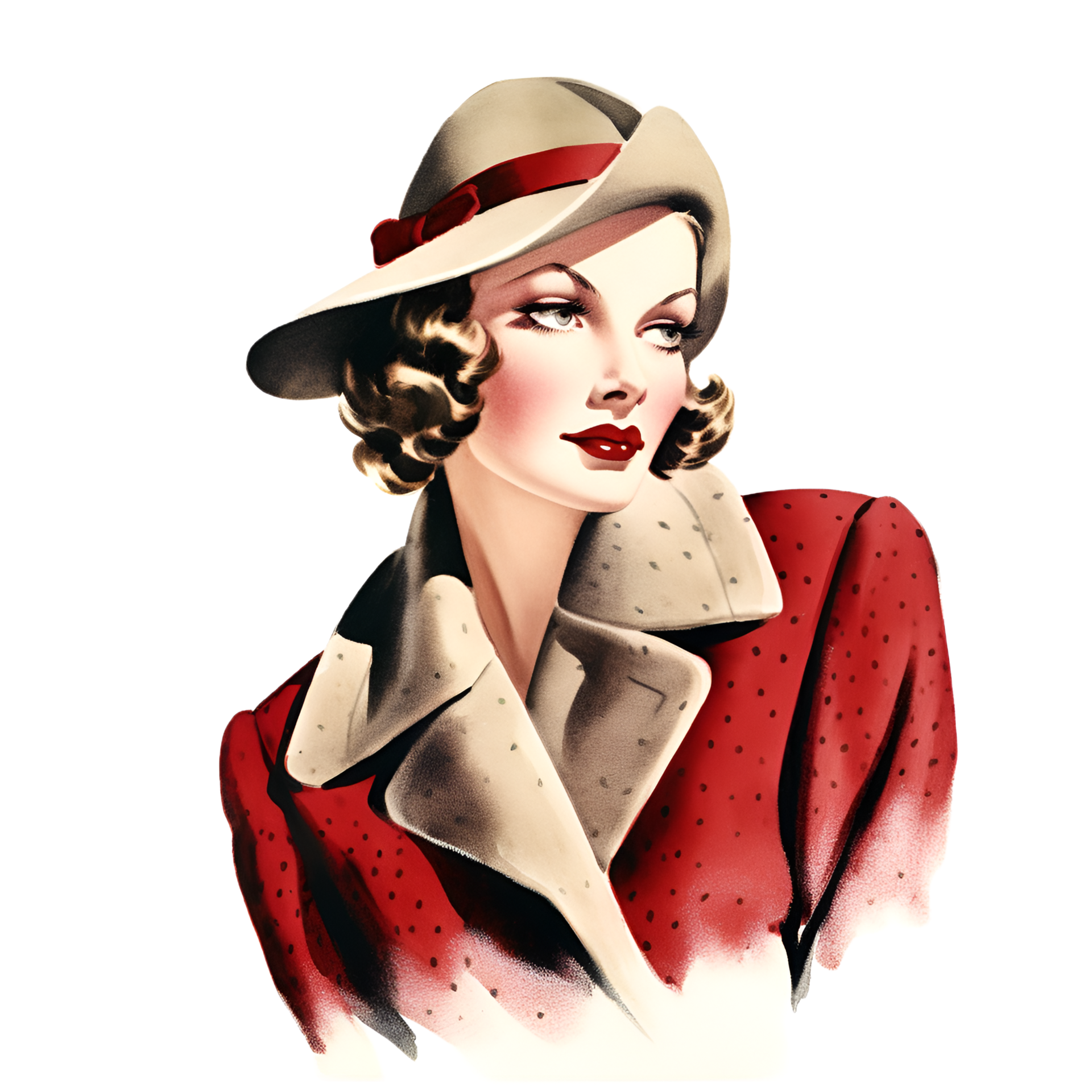The image is a detailed, vintage-inspired color illustration of a slender woman that seems to blend the essence of 1920s fashion with a 3D-rendered, airbrush style reminiscent of "Who Framed Roger Rabbit" characters. Set against a white background, the illustration portrays a porcelain-skinned woman with full, bright red lips and chin-length, wavy brown hair styled in finger waves. Her striking makeup enhances her glamorous appearance with shadowy eyeshadow, long eyelashes, and heavily arched eyebrows. 

She gazes to the right, presenting her upturned nose and refined profile. Notably, she dons a distinctive hat with an upturned brim at the front and a downturned brim at the back, featuring a red velvet hatband. Her red blazer or coat is adorned with small dark red and black dots and boasts an exceptionally broad, tan-colored lapel collar that nearly reaches her shoulders, possibly suggesting shoulder pads beneath. The jacket's vibrant strawberry hue is complemented by her rosy cheeks, completing her sophisticated look. The illustration captures her from the elbow up, with the image softly fading out towards the bottom, giving it an ethereal quality.